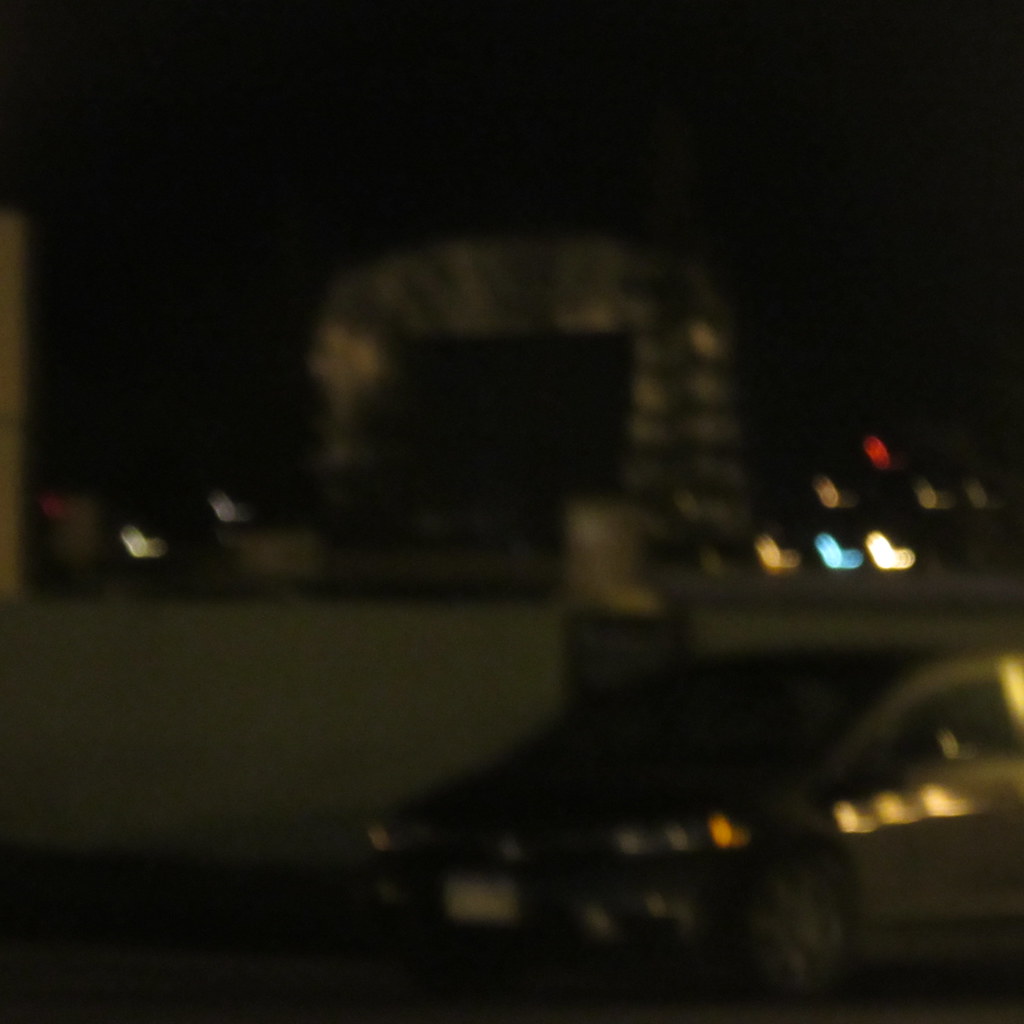This nighttime photograph, though slightly blurry due to low light conditions, captures an urban scene with the illuminated skyline of a city in the background. The focal point of the image is a mid-sized car, parked in what seems to be a parking garage, evidenced by the cement wall behind it. The car's features are discernible, including the white license plate area on the front, the shape of the headlights, and the details of the driver's side window, mirror, and tire. Light reflections highlight the edges of the car, adding depth to the composition. In the distance, a building with some windows lit up is visible amidst the ambient city lights. The background is punctuated with vibrant blue, white, and red lights, adding a dynamic contrast to the otherwise subdued scene.